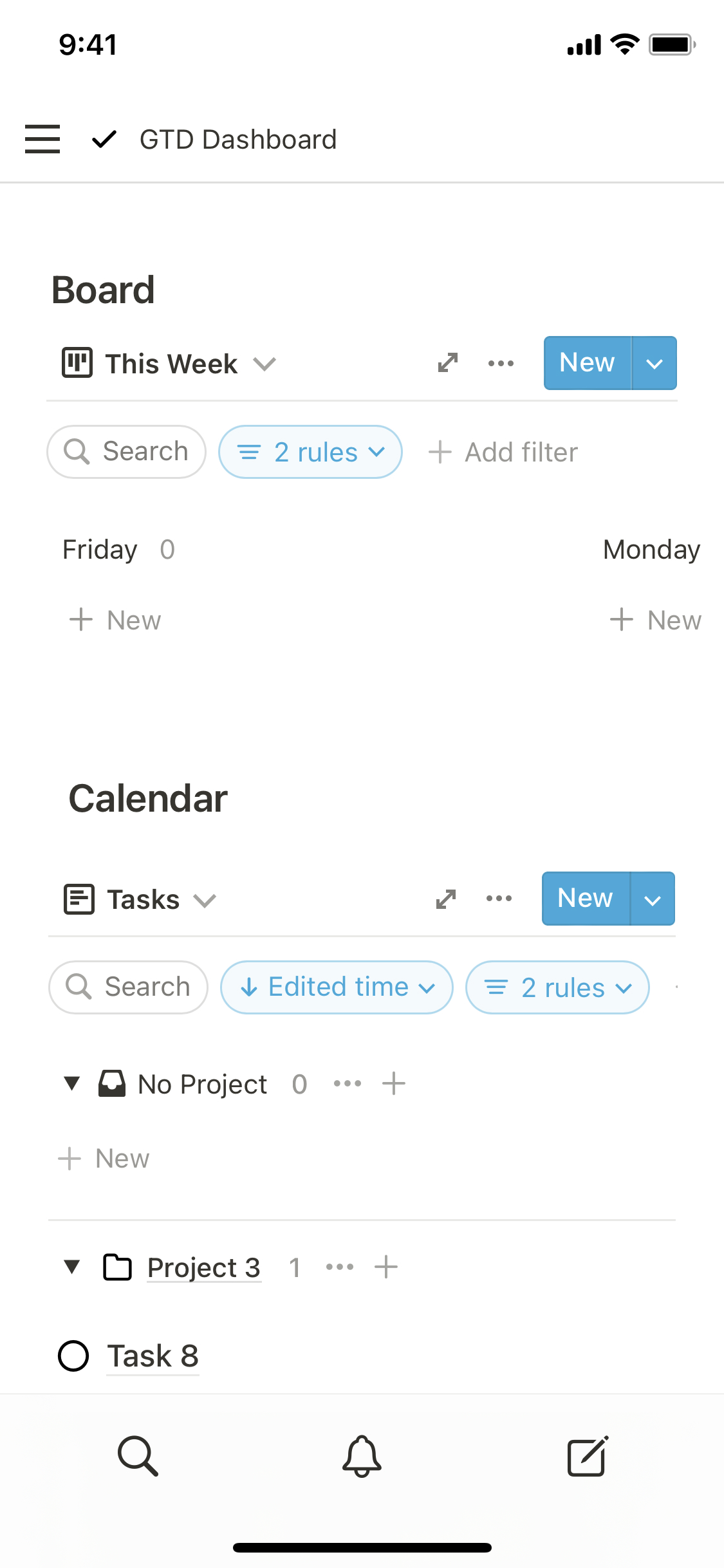The image is a screenshot of a mobile device displaying a productivity application interface, specifically the GTD (Getting Things Done) dashboard. At the top left corner of the screen, the time is shown as 9:41. On the top right corner, icons indicate a full network signal, an active WiFi connection, and battery status.

The dashboard includes several labeled sections and options. From top to bottom, these are: "BORED," "THIS WEEK," "SEARCH," "RULES," "ADD FILTER," "TASKS," "CALENDAR," "PROJECT 3," and "TASK 8." 

Additionally, there are navigation buttons at the bottom of the screen, and a smart wine glass icon is located on the left side of the interface. Toward the bottom left corner, there is a notification bell icon situated centrally at the very bottom of the screen. 

This detailed view provides an organized layout of tasks and project management features designed to facilitate workflow efficiency.